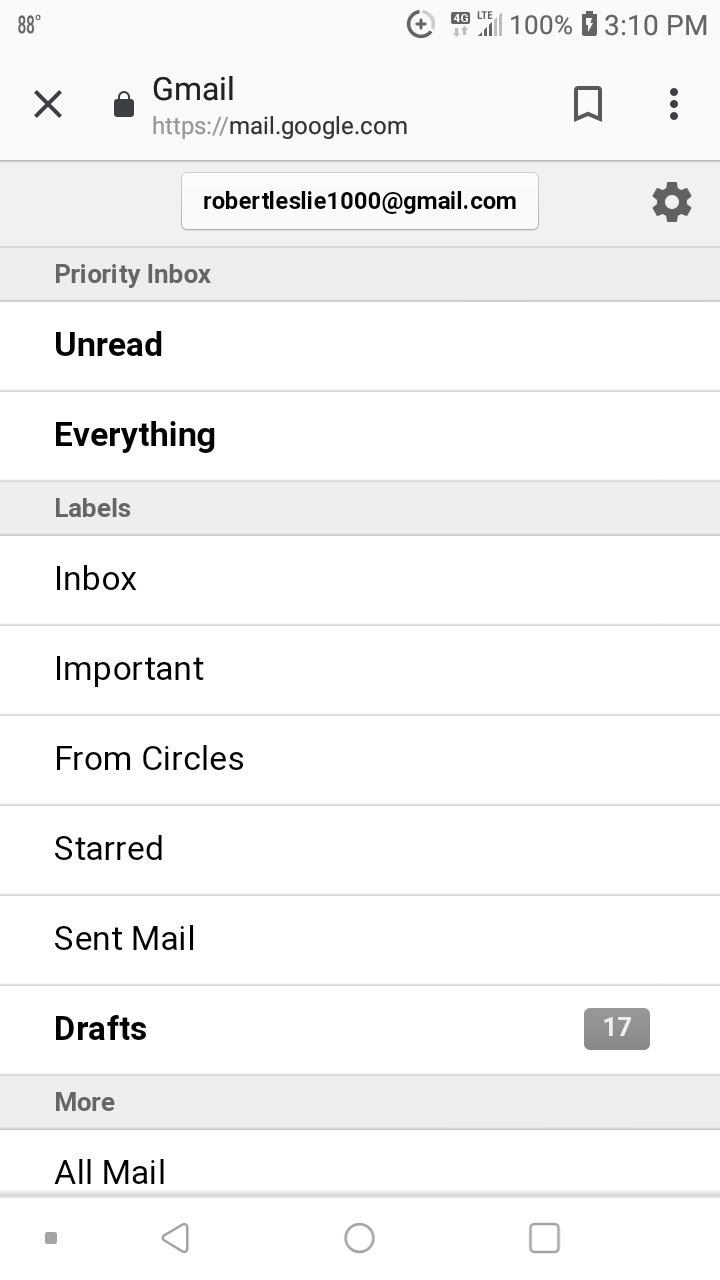**Detailed Descriptive Caption:**

The image depicts a smartphone screen displaying a Gmail inbox interface under clear weather conditions with a suggested temperature of 88 degrees. The top right corner of the screen shows the status icons, including a "+" symbol, "4G LTE" signal, a 100% battery level, and the current time of 3:10 PM. Below these status icons, the browser's URL bar is visible with the address "https://gmail.google.com". A banner is present, followed by a stack of options denoted by an ellipsis (dot, dot, dot).

The logged-in email account is "RobertLeslie1000@gmail.com", accompanied by a gear icon representing settings. The interface highlights the "Priority Inbox" with two distinct rows, showcasing unread emails and other categories. The navigation pane on the left includes various labels such as Inbox, Important, Starred, Sent, Mail, and a "More" option. Additionally, there is a gray square in the bottom left corner, with navigation symbols—a sideways triangle, a circle, and a square—indicating typical Android navigation buttons.

Overall, the interface uses a simple and organized layout to manage email efficiently, all presented within the familiar confines of a smartphone screen.